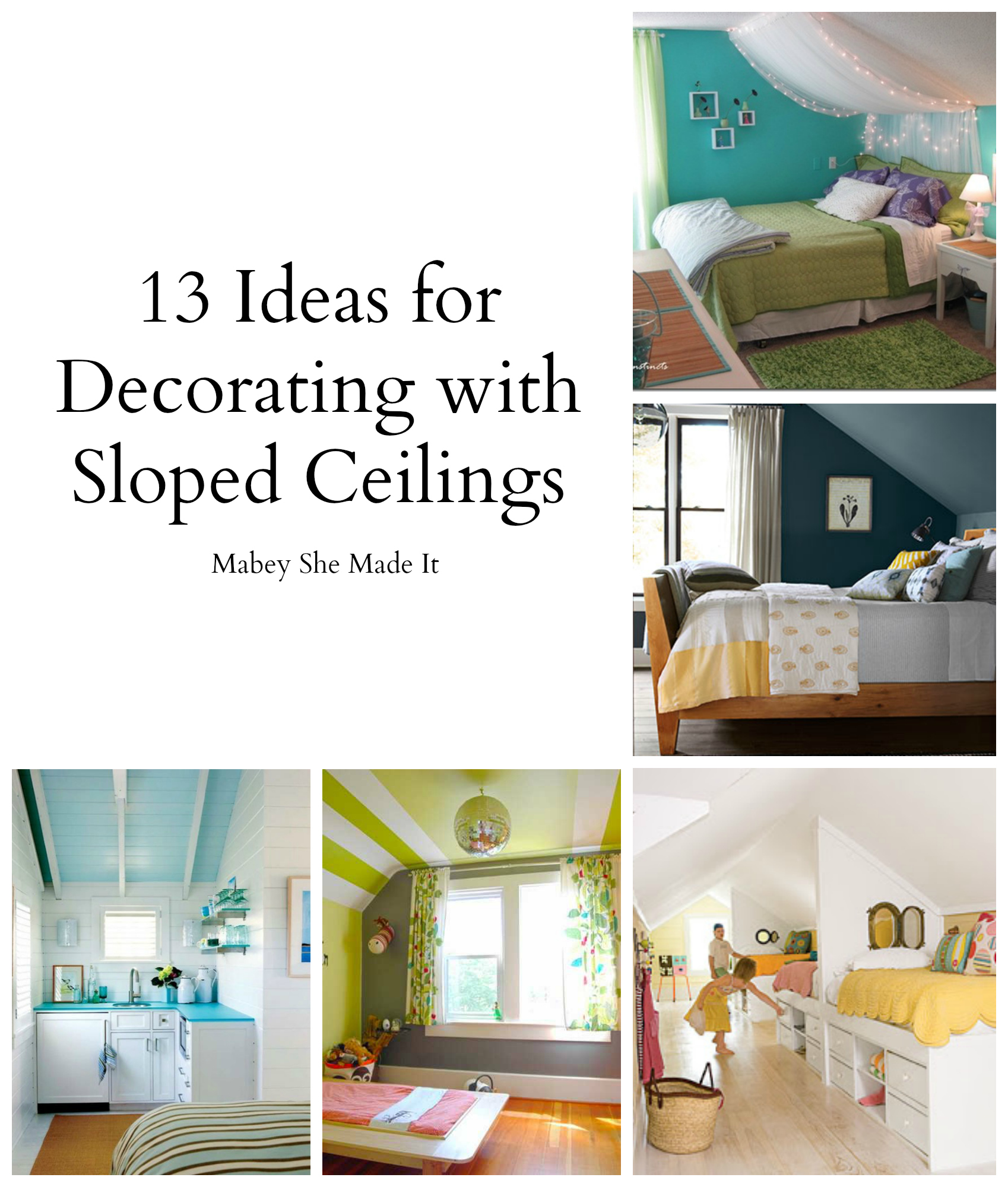This promotional image serves as a cover for a website or a magazine article titled "13 Ideas for Decorating with Sloped Ceilings" by Maybe She Made It. The layout forms an L-shape composed of five smaller images showcasing various bedroom setups, each featuring at least one sloped ceiling. The top left segment prominently displays the title in black text. The bedrooms are decorated in pastel color schemes including light blue, pink, yellow, and green. Some rooms feature combinations like green bedding with a blue-painted background, another with white and gold bedding in a blue room, while others have colorful and striped bedding. Each room showcases wood floors with unique designs and a mix of well-lit, spacious vibes. The rooms are styled with white accents, windows, and in one instance, what appears to be a small sink area. Overall, the collage emphasizes sloped ceilings' potential in creating cozy, colorful, and stylish bedroom environments.